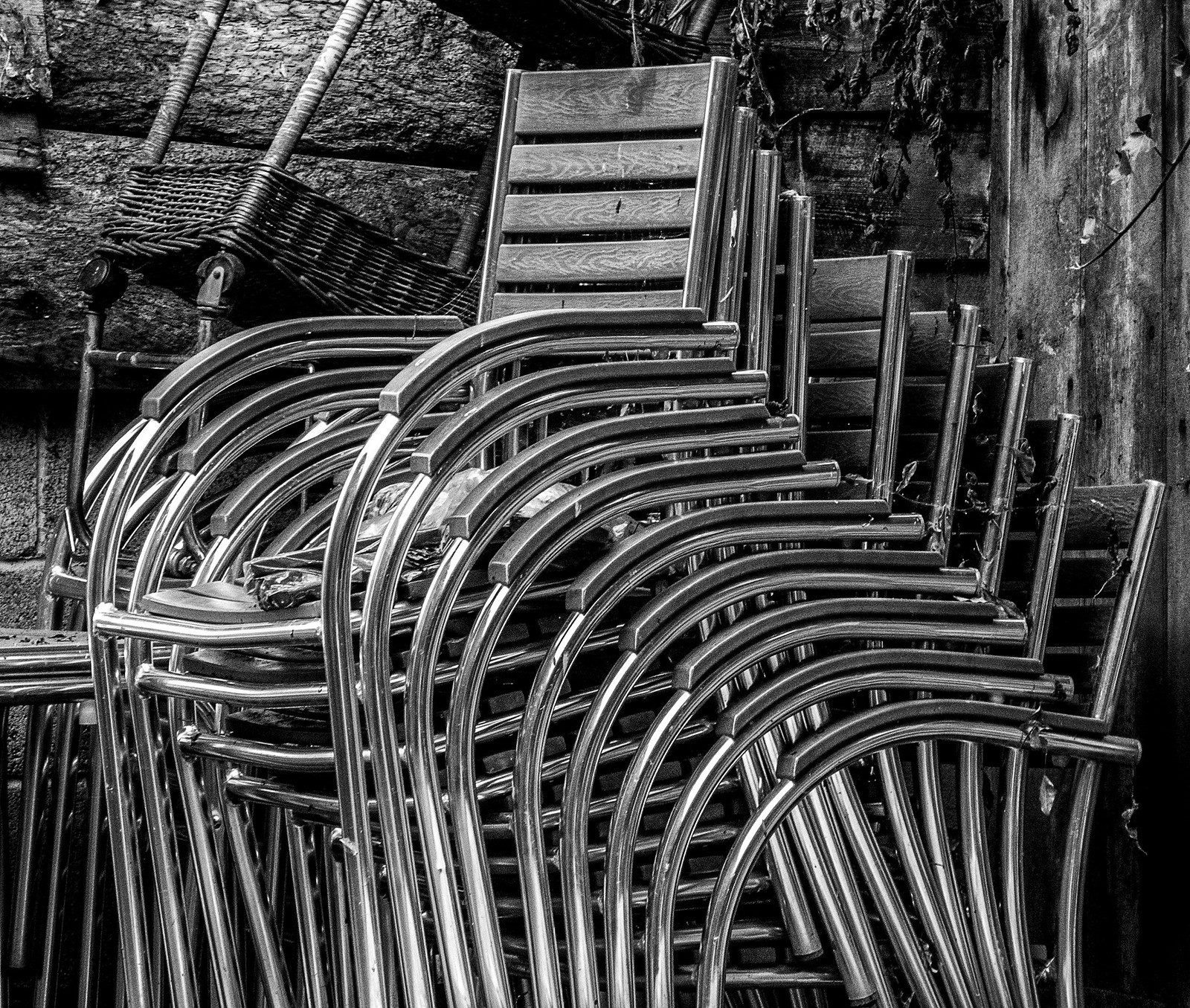This black-and-white photograph, likely taken outdoors, captures a stack of nine intricately designed chairs, creating a sense of precarious balance as they lean diagonally forward. These chairs feature horizontal wooden slats for the backrests, connected to a silver, almost chrome-like metal frame that extends to elongated front and back legs, as well as to armrests that arc gracefully downward. The chairs are compressed tightly together, forming a tall, almost topple-ready stack that commands the center of the image.

In the background, a rustic scene unfolds with a faded, jagged wooden structure partially overlaid on a wall made of concrete cinder blocks. Ivy and vines spill over the top of this structure, adding a natural element to the otherwise man-made setting. Additional stacked furniture, including what appears to be a woven basket affixed to a wheel dolly with visible black wheels, is scattered around, heightening the sense of organized disarray. The backdrop also features elements like a possible brick wall and worn surfaces, contributing to the photograph's layered, textured ambiance. This rich composition suggests an outdoor patio, possibly of a restaurant, filled with an eclectic mix of objects, both organic and industrial.